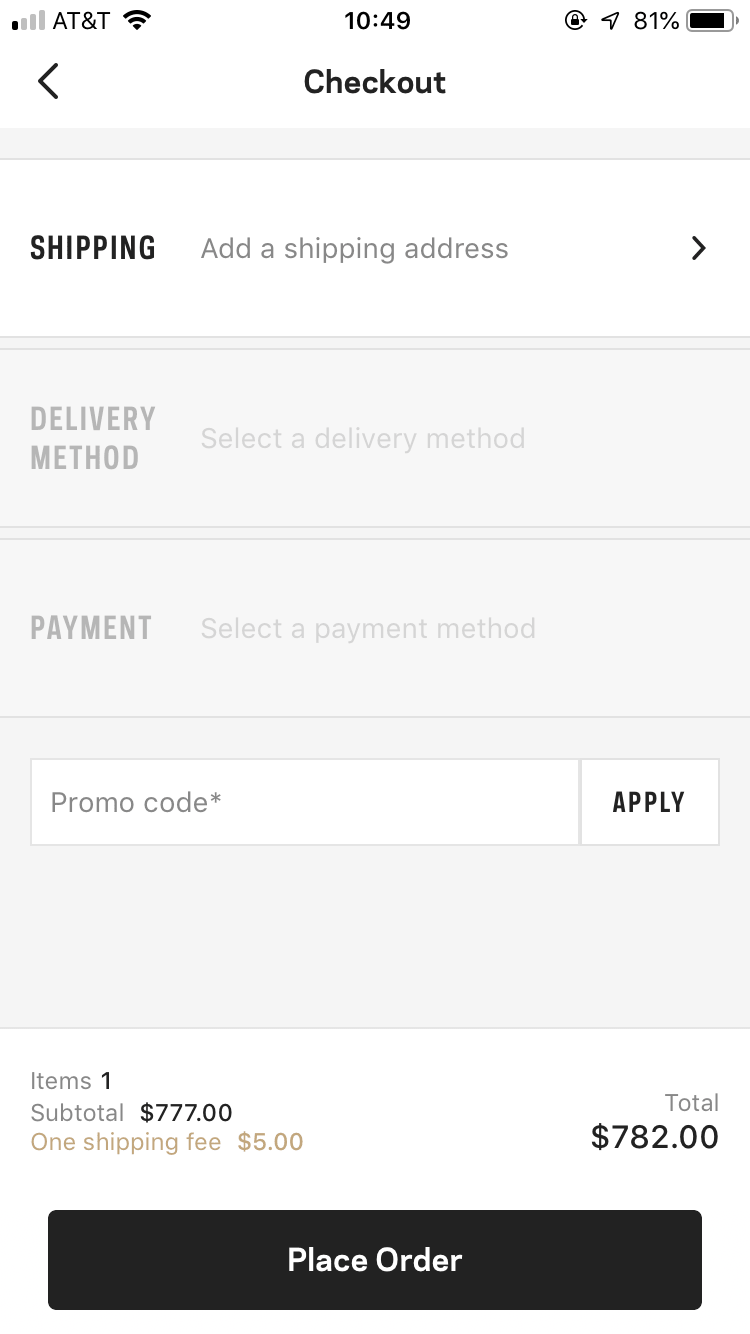The image showcases a checkout screen for an app displayed on a smartphone. At the very top of the screen, the phone's status bar is visible, indicating network signal strength, an AT&T carrier label, Wi-Fi connectivity, the current time, and a battery level indicator. 

Directly below the status bar, the header "Checkout" is prominently displayed in black and white. The first section beneath the header is labeled "Shipping," featuring a clickable box prompting the user to "Add a shipping address." 

Next, there is a section titled "Delivery Method," which instructs the user to "Select a delivery method." The subsequent section, "Payment," similarly prompts the user to "Select a payment method."

Further down, there is an input field labeled "Promo Code," accompanied by an "Apply" button. 

At the bottom of the screen, the order summary is presented: it states "Items: 1", provides a subtotal of "$777," adds a "Shipping Fee: $5," and calculates the "Total: $782."

The screen concludes with a prominent, black "Place Order" button at the bottom.